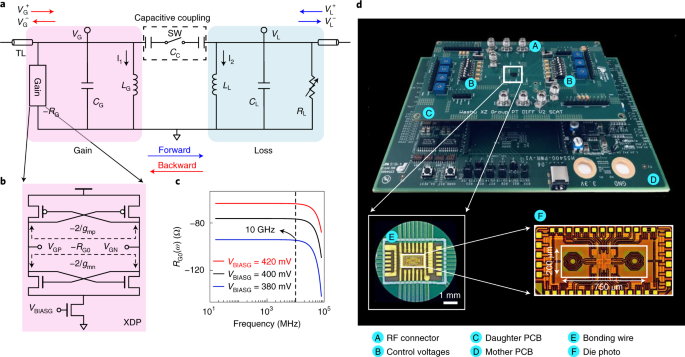The image consists of two main sections: a detailed electrical schematic on the left and a complex diagram of computer hardware on the right. The left side features a drawing labeled "Capacitive Coupling," depicted with pink, white, and blue elements, and annotated with terms such as "forward," "backward," and "loss," alongside various numerical data. The schematic illustrates the intricate paths of electrical currents and connections. On the right side, the image displays a detailed view of a motherboard, highlighting both a smaller daughter PCB mounted on a larger mother PCB. The components are labeled with letters A to F, identifying parts such as the RF connector, control voltages, and bonding wire. The motherboard appears gold-plated in sections, featuring blue connectors and an enlarged circular detail marked "E." Overall, this image provides a comprehensive visualization of both the theoretical and physical aspects of the electronic components.